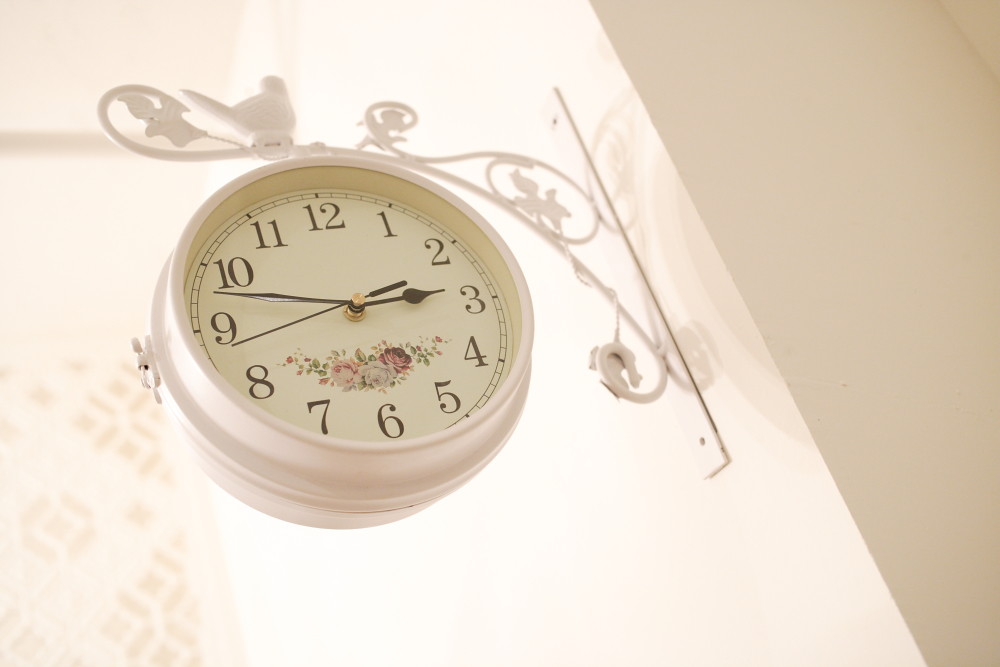This photograph, taken indoors at an upward angle, showcases a detailed decorative wall clock mounted in someone’s living room. The clock is affixed to a white wall via an ornate metal bracket featuring vine-shaped designs and a perched bird. This bracket, comprised of elegant swirls and curves, extends vertically, giving a sophisticated look. The round clock itself hangs from this bracket and is encircled by a thick white frame. The clock face is also primarily white with a slight cream hue and is adorned with a cluster of three pink roses along with their leaves, located above the number six. The black numbers marking the hours are clearly visible, and the minute markers encircle the face without numeric labels. The hour and minute hands are black, with the hour hand ending in a spade-like shape, while the sweep second hand is also black and slightly shorter than the minute hand. In the background, the right edge of the image shows a neighboring wall cast in shadow, contributing to the depth and composition of the photograph. The overall setting, including the hint of another wall with cream-colored geometric patterns, frames the decorative clock elegantly against the corner of this white-painted room.